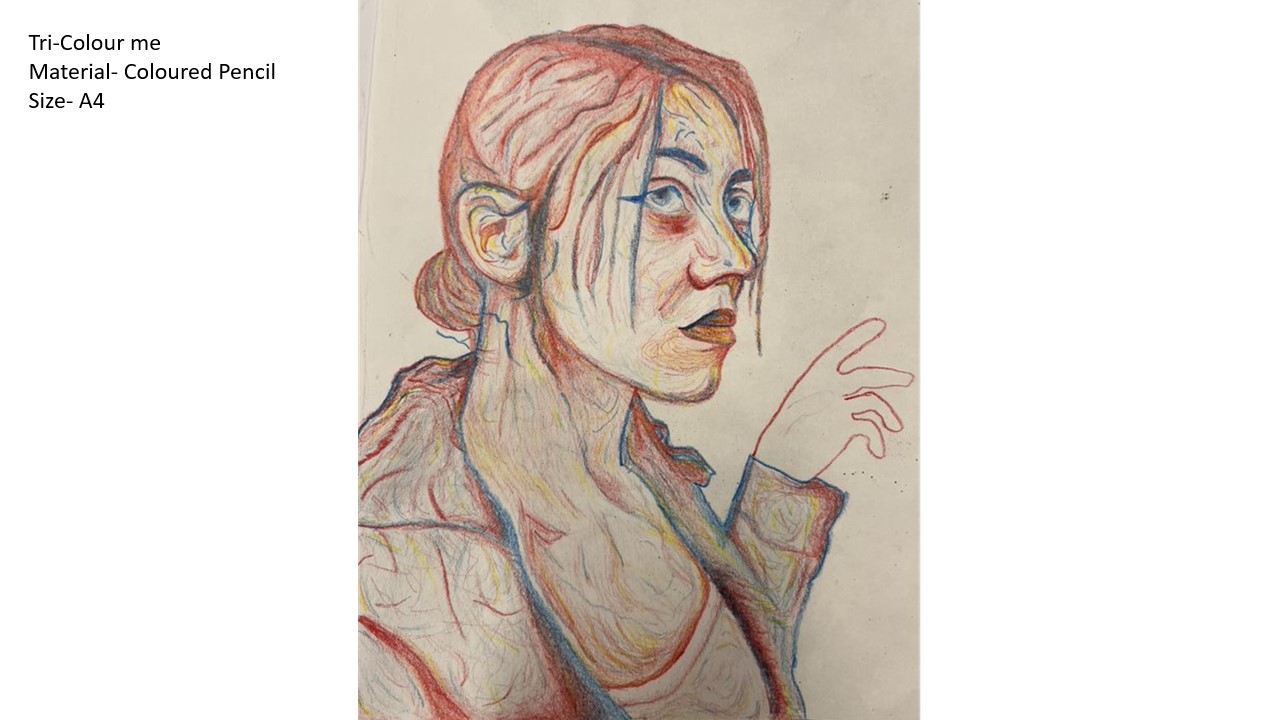This is a colored pencil drawing on an A4-sized sheet of plain white paper, named "Try Color Me." The image features a woman in a three-quarter profile angle, predominantly displaying her right profile with her hair, a striking red, pulled back into a ponytail at the base of her neck. Wisps of hair escape, framing her cheek. She has a rather severe facial expression, enhanced by the vivid use of colors: blue makeup around her eyes, with red and yellow accents on her face, including around her nose and under her eyes. The woman is dressed in a white shirt trimmed with red and layered with a jacket. Her left hand, not fully detailed and lacking the thumb, is raised. Various colors, including unexpected touches of blue in areas where they traditionally wouldn’t go, add depth and intrigue to the composition. The background is a plain white, emphasizing the bold coloration of the subject.